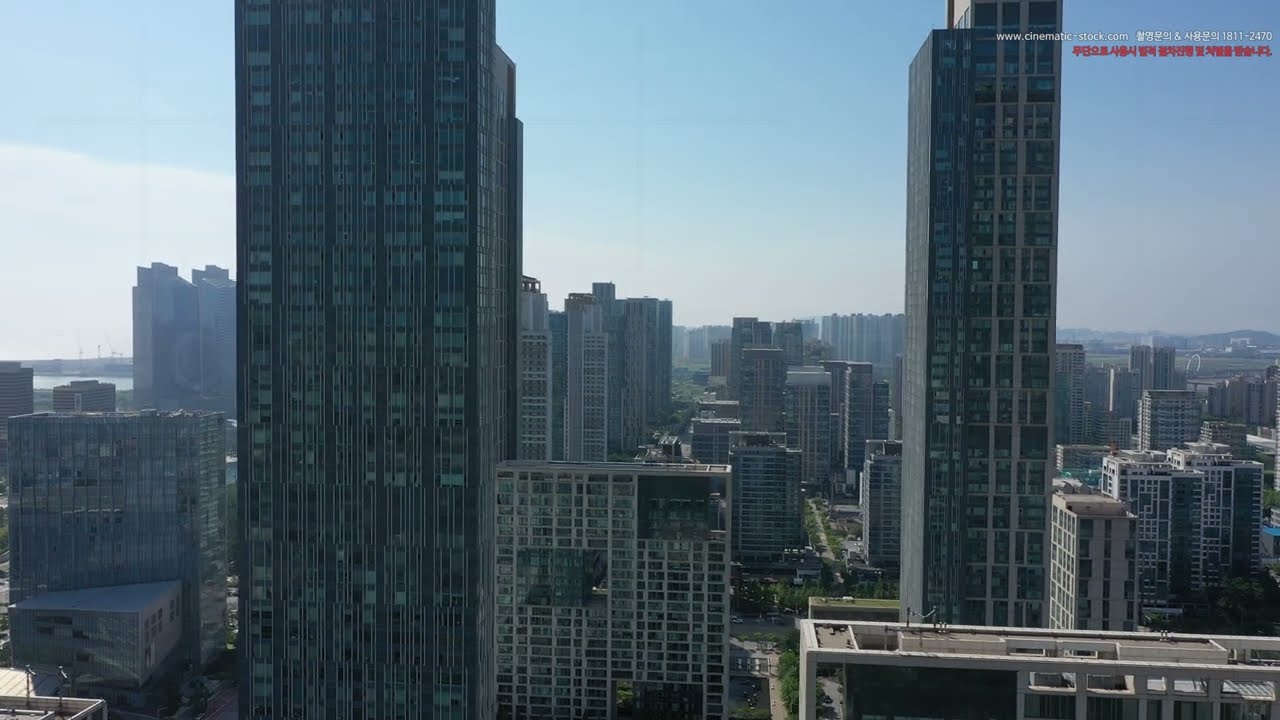This high-definition photograph captures a bustling cityscape in a large metropolitan area, likely in a warm climate due to the prevalence of white buildings. Dominating the center are two tall residential buildings—one on the left, which appears thicker, and one on the right, which features visible patios. The buildings are modern, constructed from steel and metal with numerous windows, contributing to the sleek, urban aesthetic. Interspersed between these central buildings are various high-rises of varying heights, suggesting a financial district with banks and business parks. The background reveals a bright blue sky with white clouds, adding to the vibrant atmosphere. Notably, the photograph includes text in the upper right corner: “cinematicstock.com” in white, alongside additional Chinese characters, indicating the image's origins or usage rights. To the left, a body of water, potentially a lake or ocean, is visible, balancing a small mountainous area to the right—both adding natural elements to this urban tableau.